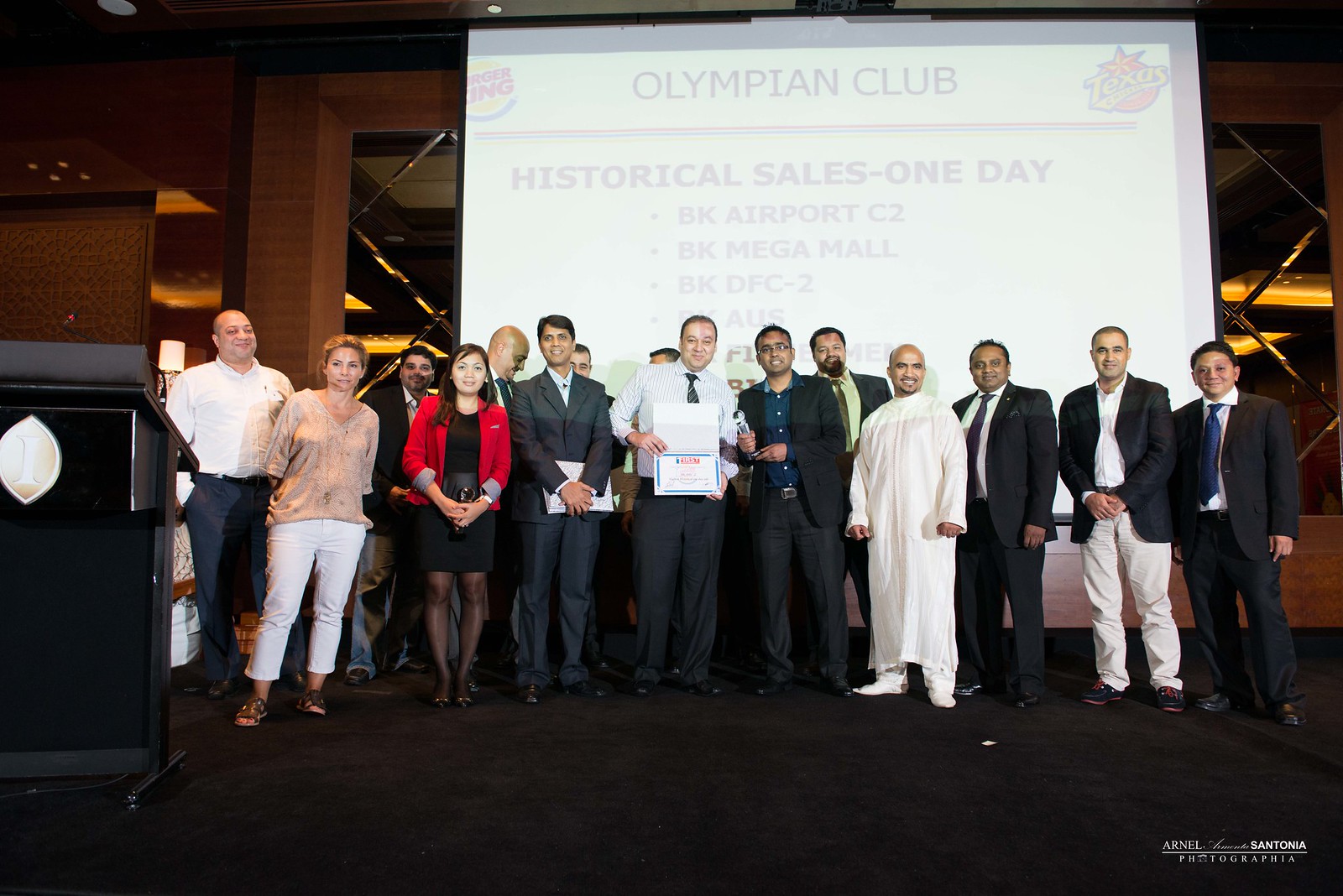In a spacious conference room with a black carpet and brown trim, a celebratory business meeting is taking place. Approximately 12-15 well-dressed men and women are gathered on stage, all smiling and holding a plaque. The overhead projector displays significant text, including "Olympian Club," "Burger King," "Texas," and "Historical Sales One Day." The event appears to honor exceptional sales achievements at various Burger King locations: BK Airport C2, BK Mega Mall, and BKDF C2. The attendees, likely Burger King sales team members behind these accomplishments, stand against a backdrop that signifies a formal and triumphant occasion.